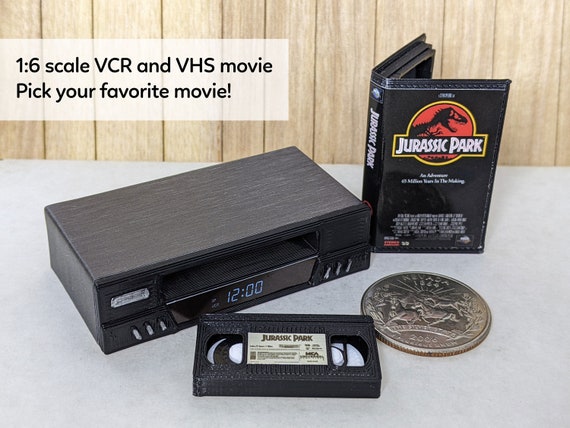This image features a miniature display on a light gray table against a backdrop of vertical light brown wooden slats. On the upper left, a white rectangle with black text reads, "1 to 6 scale VCR and VHS movie. Pick your favorite movie!" Dominating the scene is a very simple, rectangular, black mini VCR, meticulously 3D-printed with a wood grain texture top, and a small digital clock display showing "12:00" with three buttons on each side. Resting in front of the VCR is a 3D-printed miniature VHS tape marked by a white label with "Jurassic Park" written on it, nestled between two viewports. To the right of the VCR stands the VHS case for Jurassic Park, prominently displaying its iconic cover art: a black background with a red circle outlined in yellow and a skeletal dinosaur image. For scale, a Nevada State U.S. quarter from 2006 lies beside the tape, illustrating the tiny dimensions of this nostalgic setup.